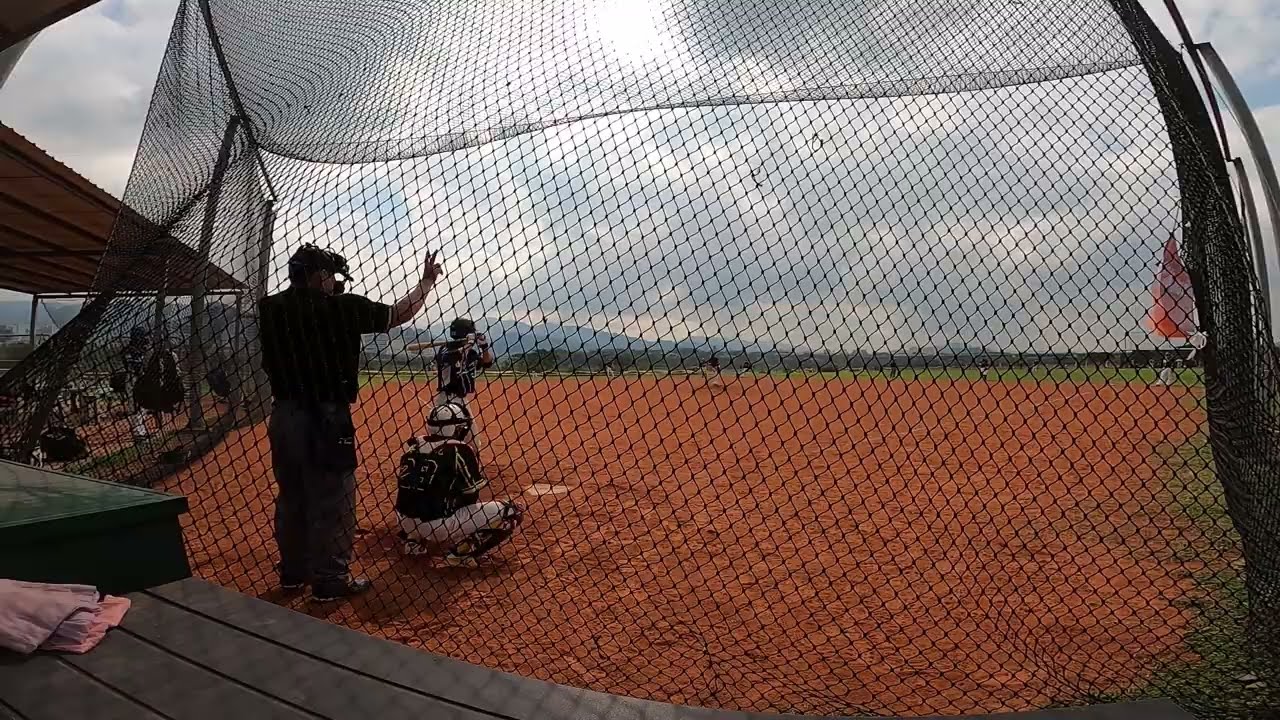In the image of a Little League baseball game, the scene unfolds on a baseball diamond with distinctive red dirt and patches of green grass in the background. The sky above is overcast, with clouds obscuring the sun, creating a muted light over the field. At the center of the image, viewed through a fish-eye lens, a large protective net stands behind the umpire, adding a subtle curvature to the scene.

The umpire, dressed in a black shirt and black pants, stands upright with a mask on his face, extending his right arm to signal with two fingers in the air. Positioned in front of him is the catcher, fully equipped with white pants, white helmet, mask, and other protective gear, squatting in anticipation. Directly before the catcher, a batter stands at home plate, bat poised behind him, focusing intently on the impending pitch.

To the left side of the scene, some onlookers gather, possibly near a dugout area. In the lower left corner, a set of steps, possibly part of a stand, is visible with a towel draped over it. The entire setting is viewed from near the stands behind the pitcher and the umpire, capturing the intricacies of this spirited moment on the brownish-orange field.